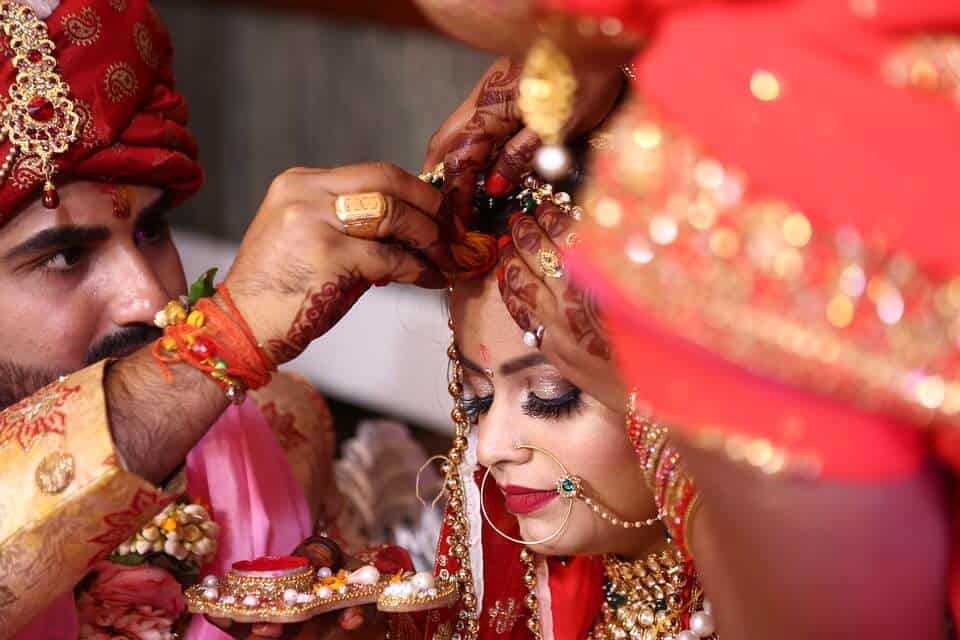In this vibrant rectangular image, only the heads of two individuals, possibly of Indian or South Asian descent, are visible, as they prepare for a ceremonial event. The man on the upper left is adorned in a richly decorated outfit: a red turban with cascading gold accents, a gold-colored shirt with red floral designs, and a pinkish scarf. His arm, clothed in a gold sleeve with red decorations and adorned with numerous bracelets, partially obscures his face as he places a decorative item on the woman's forehead. He also wears a prominent rectangular gold ring. The woman, positioned centrally in front of the man, has her eyes closed and appears serene. Her appearance is equally adorned with opulent jewelry, including extensive gold beads and two large hoop nose rings connected by gold chains. Her dark red lipstick contrasts with her bronze eyeshadow and long black eyelashes. They both appear deeply engaged in what seems to be a traditional ceremony or festive ritual.